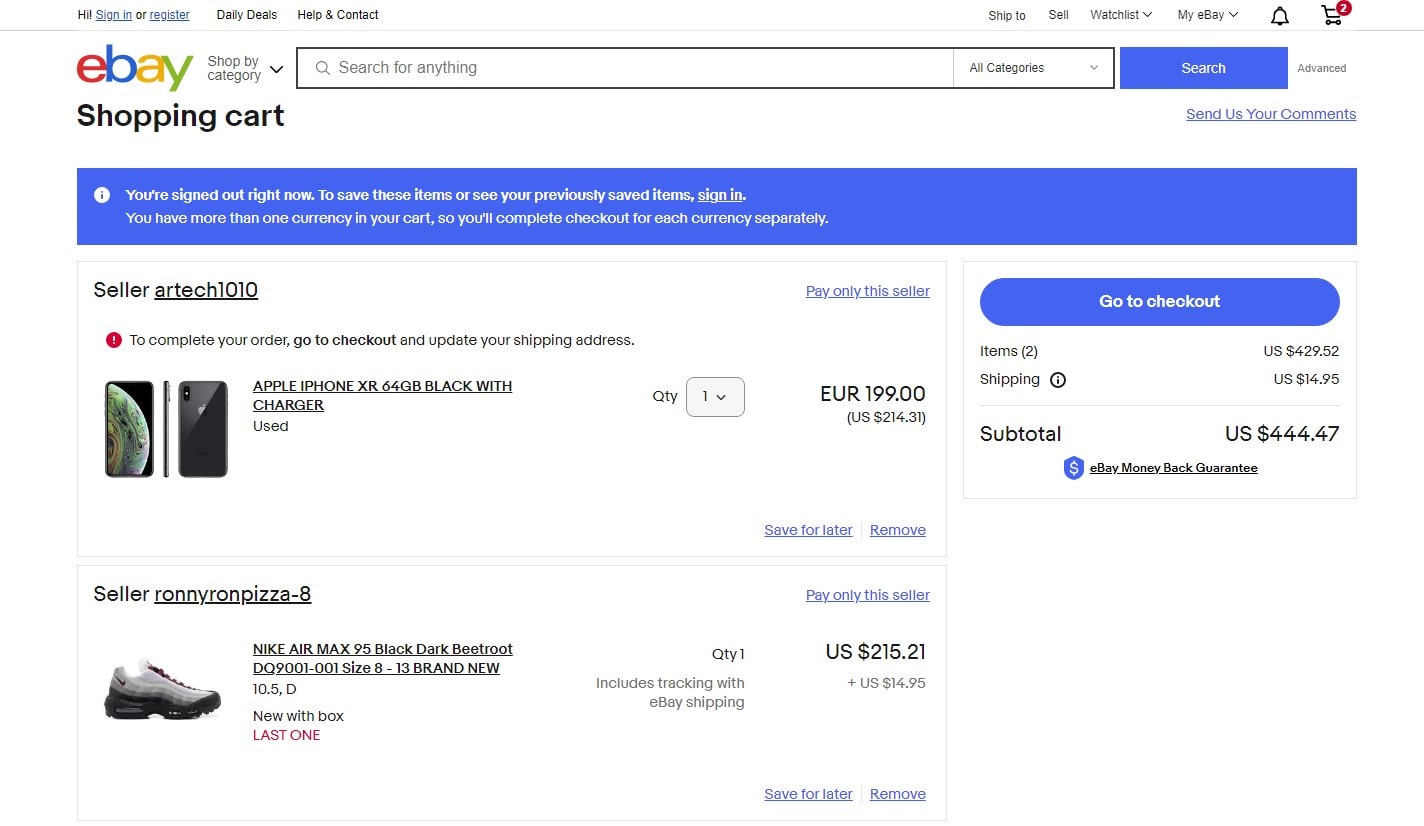Screenshot of an eBay shopping cart displaying two items:

1. **Apple iPhone XR, 64GB, Black with Charger**
   - Price: EUR 199 (approx. USD 214.31)
   
2. **Nike Air Max 95, Black/Dark Boot Root, Sizes 8-13, Brand New in Box**
   - Price: USD 215.21
   - Shipping: USD 14.95

**Subtotal of Items: USD 429.52**

**Total Shipping Cost: USD 14.95**

**Overall Subtotal (Including Shipping): USD 444.47**

The screenshot provides a detailed view of the eBay shopping cart, summarizing the total costs for both items without a specified date.